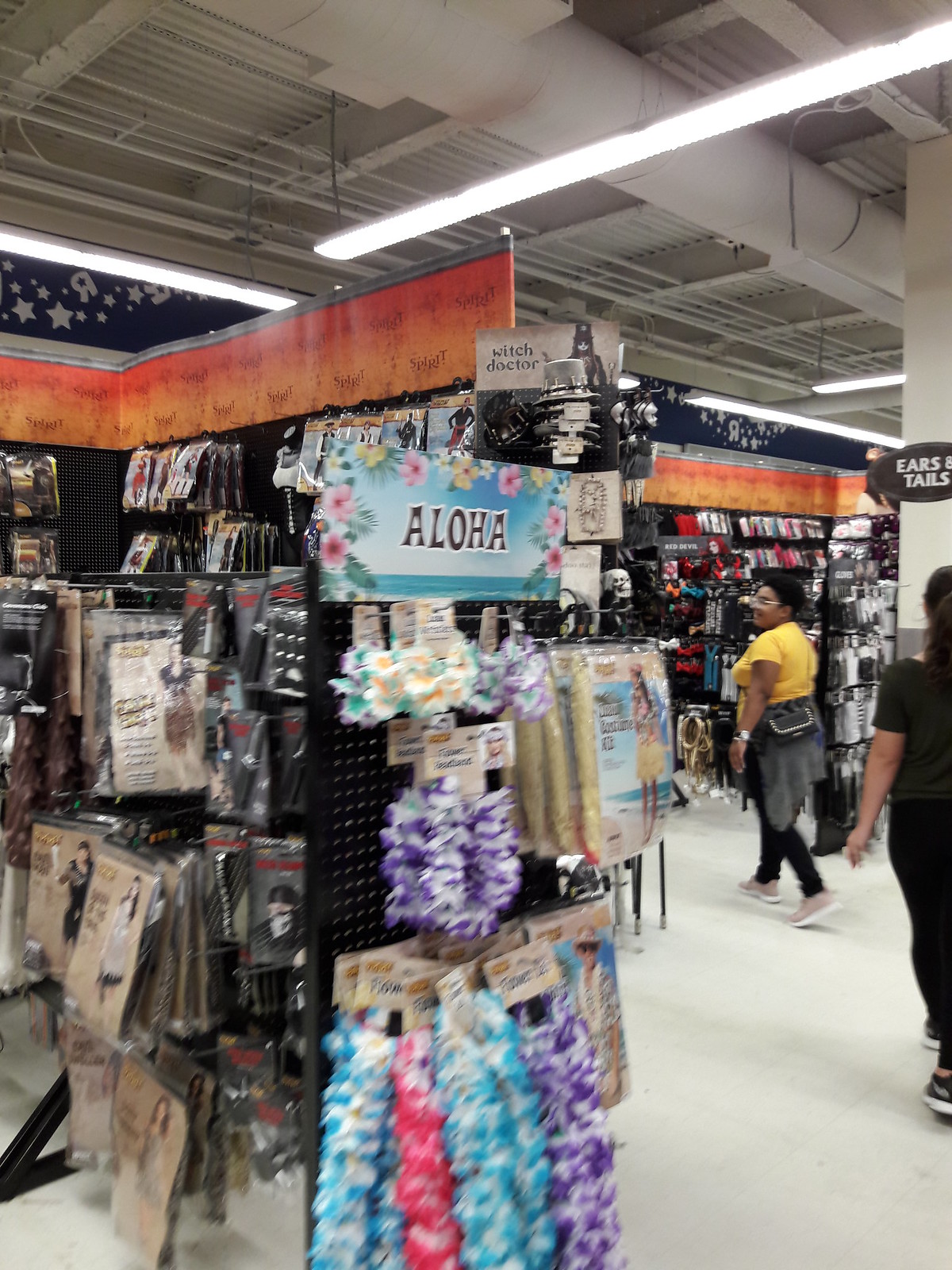The image captures the vibrant interior of a party supply store, likely a Zurcher's or a similar retailer. The store is filled with various party supplies, with an array of decorations visible along a sidewall. Among the shoppers, two women can be seen: one dressed primarily in black and the other wearing black pants and a yellow shirt. On one sidewall, a sign reading "Ears and Tails" is prominently displayed, indicating a selection of dress-up accessories, possibly for Easter-themed events. Nearby, another section labeled "Aloha" showcases colorful leis and other Hawaiian-themed party essentials. The store also features an assortment of costumes and additional party decorations, contributing to the lively and festive atmosphere.